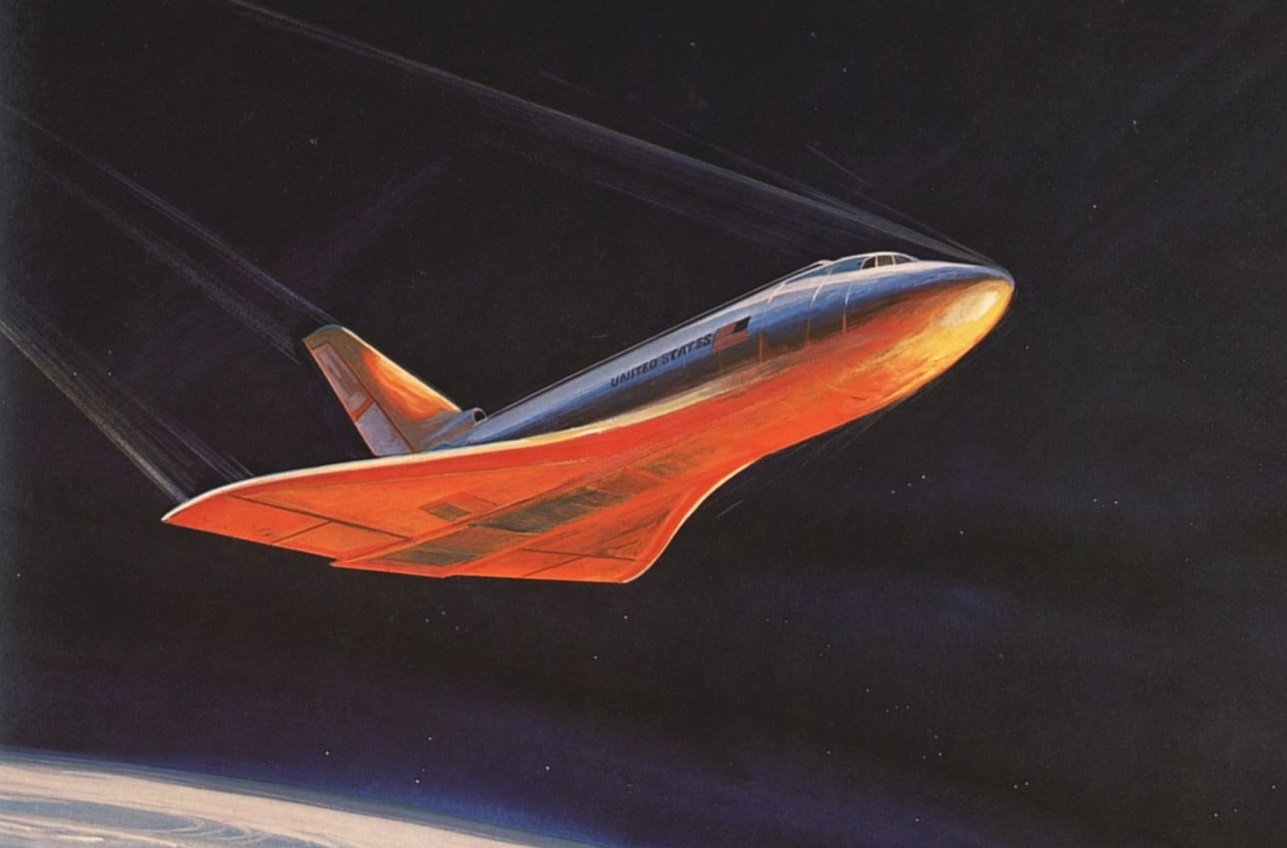This graphic illustration captures a stylized spacecraft resembling the iconic space shuttle during its dramatic reentry into Earth's atmosphere. The scene is rendered from a perspective beneath the shuttle, highlighting its underside, which is aglow with a cherry-red hue indicative of intense heat from reentry friction. The dark blackness of space forms the backdrop, sparsely populated with stars. The shuttle is depicted at a roughly 45-degree angle, nose pointed upwards, with its tail fin trailing behind. Streaks depicting the shuttle's rapid descent accentuate the sense of motion. The American flag and the words "United States" are prominently displayed on the shuttle's side. In the lower left-hand corner of the image, a small portion of Earth is visible, suggesting the shuttle's proximity to home. The faint glow around the Earth and the stylized heat effects on the shuttle create a vivid contrast against the emptiness of space, underscoring the peril and precision involved in the reentry process.